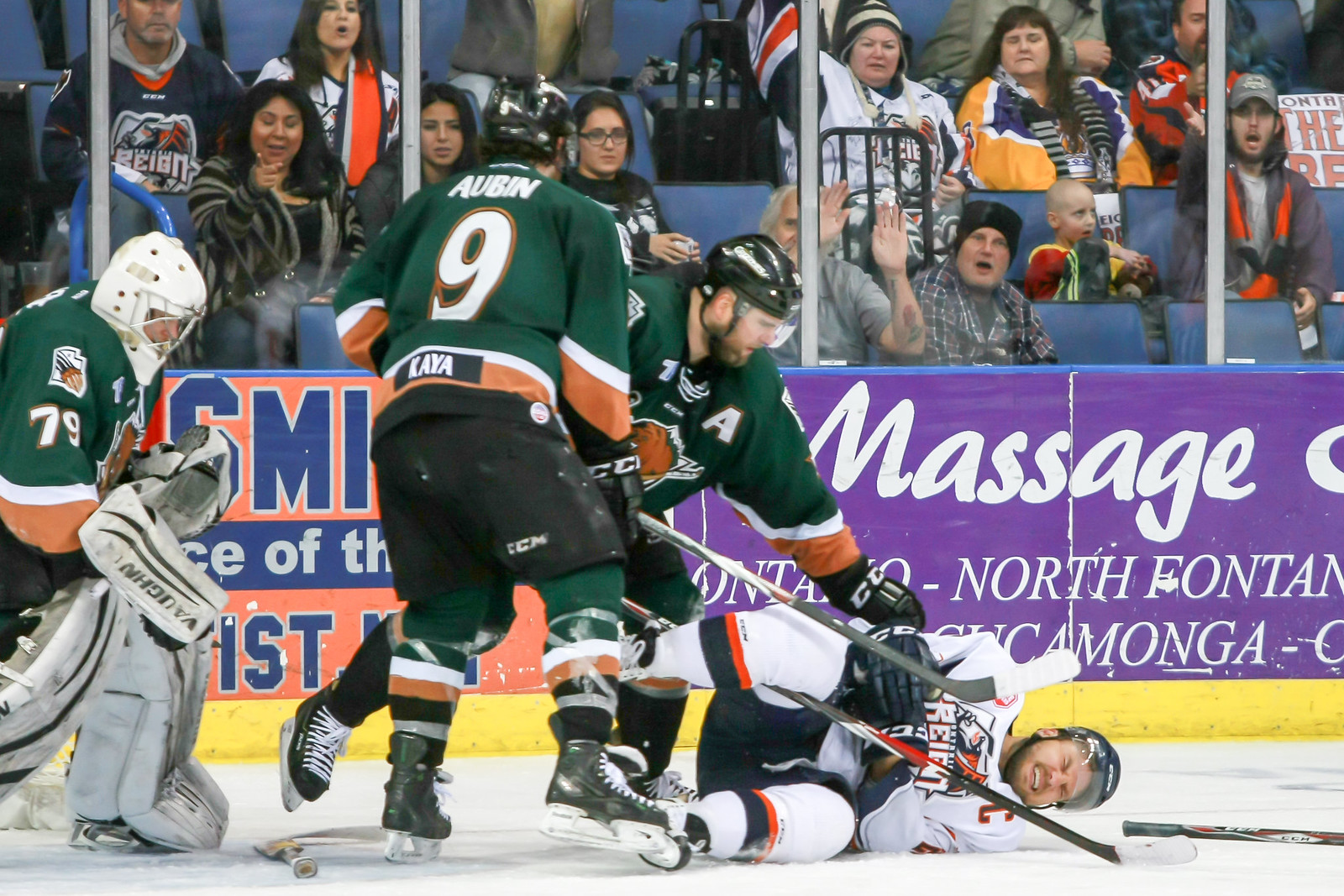This image captures an intense moment in a hockey game featuring players from two distinct teams. The green team's players, identifiable by their green jerseys accented with black and gold, are prominently featured. Three of them are standing upright: one wearing an "A" for assistant captainship and another with the number 9 jersey. The goalie, adorned with a white mask and thick white pads, is positioned on the left side of the image, facing towards the right.

On the ice, a player from the opposing team, dressed in a white jersey with orange and blue accents, lies on his left side, grimacing in apparent pain. He wears the letter "C" on his right shoulder, marking him as the team captain. His right leg is raised while his left is pressed against the ice. His hockey stick is partially visible on the right side of the image. The scene is set against a vibrant backdrop of a crowd in the bleachers, peering through the glass. An advertisement with a purple banner that reads "massage" is also visible, adding to the lively atmosphere of the rink.